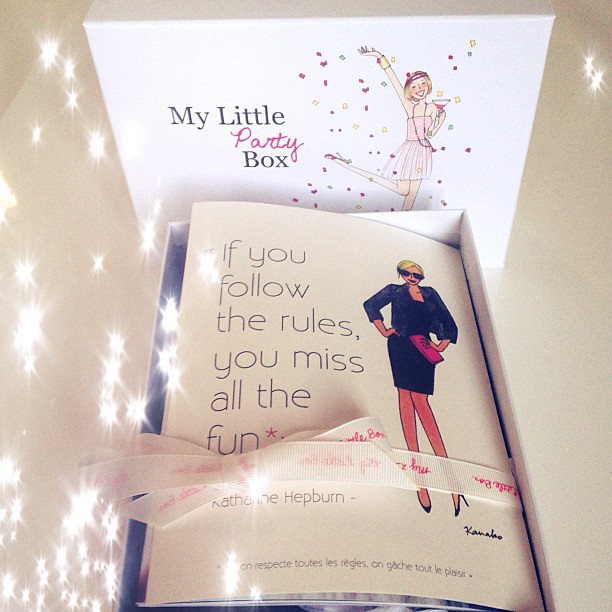The image depicts an open "My Little Party Box," with its lid standing upright as the backdrop. The box lid features an illustration of a pixie doll or cartoon woman in a cocktail dress, throwing confetti, with a martini glass filled with red liquid in one hand. The lid text reads "My Little Party Box," with "My Little" and "Box" in black and "Party" in pink. The scene has a light lavender background with superimposed white stars or glitter.

Inside the box is a collection of papers or booklets, neatly wrapped in a white ribbon. The visible top sheet of these papers displays a quote, "If you follow the rules, you miss all the fun," attributed to Catherine Hepburn. Another notable item within the box is a drawing by artist Ken Kanar-Kamaho, depicting a blonde woman with sunglasses, wearing a blue long-sleeve top, a black skirt, and heels. The overall presentation suggests a lively party theme, emphasized by the vibrant illustrations and celebratory motifs.